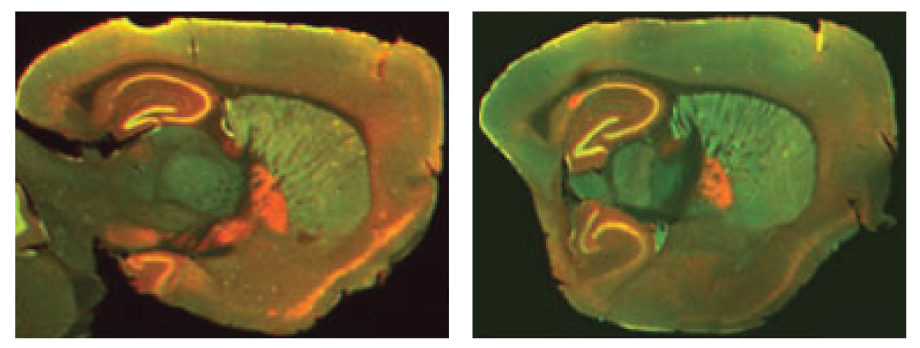The image features two horizontal rectangular photographs of handmade ceramic bowls, placed side-by-side against a dark background. The bowl on the left showcases a green base with an orange figure extending into the center, and the sides are in varying hues of brown and green with a regular edge. A brown cutout figure is positioned behind this bowl. The bowl on the right, although similar in size, differs in shape. It primarily displays green walls and a very green bottom, accented by an orange-headed figure with a few brown, swirly designs. Both bowls, while sharing similarities like color schemes of green, brown, and orange, exhibit distinct shapes and patterns.